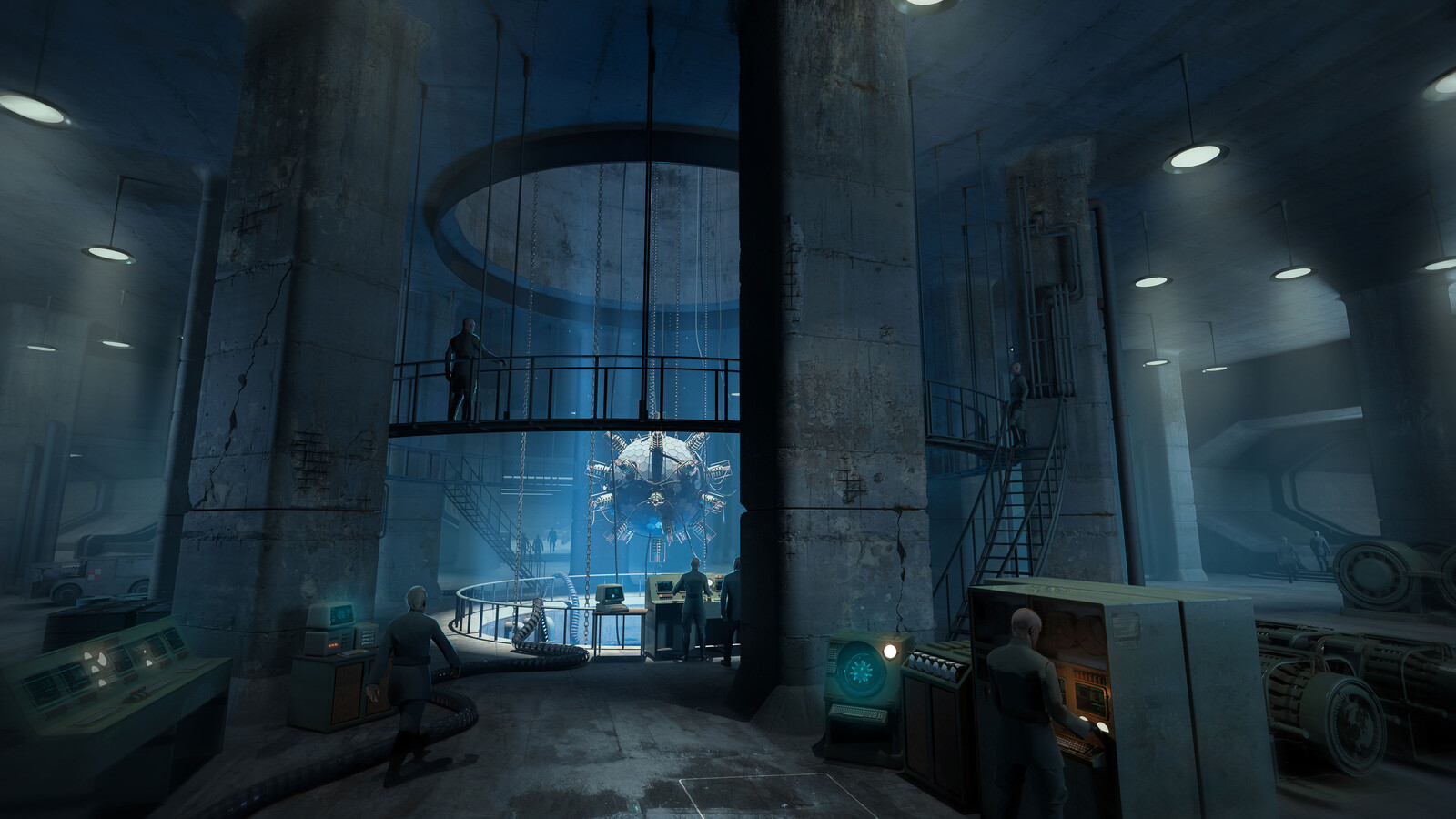This image is a detailed color illustration, likely created for a video game or animation, depicting a cavernous, futuristic laboratory set within a large, dark, cave-like space with tall ceilings supported by cement pillars. The scene is illuminated by recessed lights overhead, accentuating the high-tech atmosphere. At the center of the lab, there is a prominent, round structure with a clear glass enclosure at the top, containing a large, hanging orb that resembles a spacecraft or satellite. The floor appears to be cement, and technology abounds throughout the space, with multiple control panels featuring lights and controls. Several figures are dispersed across the laboratory; one individual is positioned in front of a control panel on the lower right, facing away from the viewer, while others are interacting with similar panels on the left side and upper levels. The walk-around platform surrounding the central structure provides a vantage point for observing the orb below. The overall scene is vivid and meticulously detailed, with an emphasis on the advanced technological setting created by artist Charles E.J. Downman in the work titled "Command and Control."